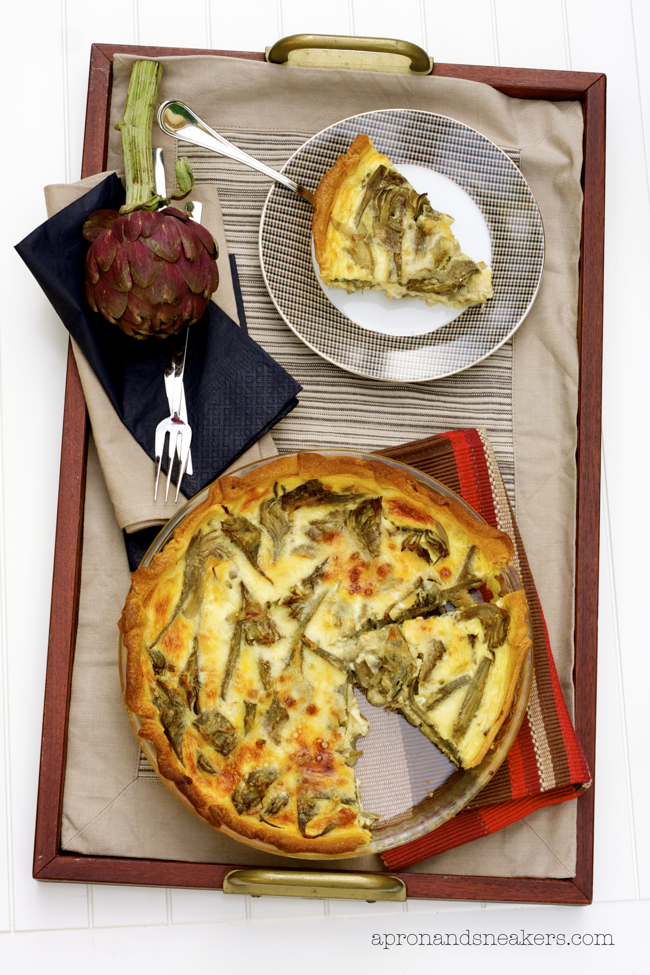The image showcases a beautifully styled food display, likely something found in a gourmet food magazine. Central to the composition is a dark walnut wooden tray with elegant brass handles, situated on a white shiplap surface. The tray is lined with a tan cloth and features a clear glass pie pan containing a savory quiche. This quiche has a delightful golden crust with visible asparagus and cheese on top, suggestive of a rich, egg-based dish. 

In the top section of the tray, there is a sophisticated black and white striped plate with a slice of the quiche atop a silver serving fork. Below this, the full quiche occupies most of the scene, positioned on a striking brown, red, maroon, and tan striped napkin. To the left of the quiche, a beautifully folded black napkin sits atop a cream-colored one, adorned with a silver fork and knife and crowned by a vivid purple artichoke with a green stem.

The setup is further enhanced by a polished presentation: black and brown folded napkins add a refined touch. At the bottom of the image, the URL "apronsandsneakers.com" is subtly printed, providing a hint of the source. The meticulous arrangement of the elements against the white, slatted wooden backdrop underscores the elegance and culinary allure of the dish, making it an inviting feast for the eyes.